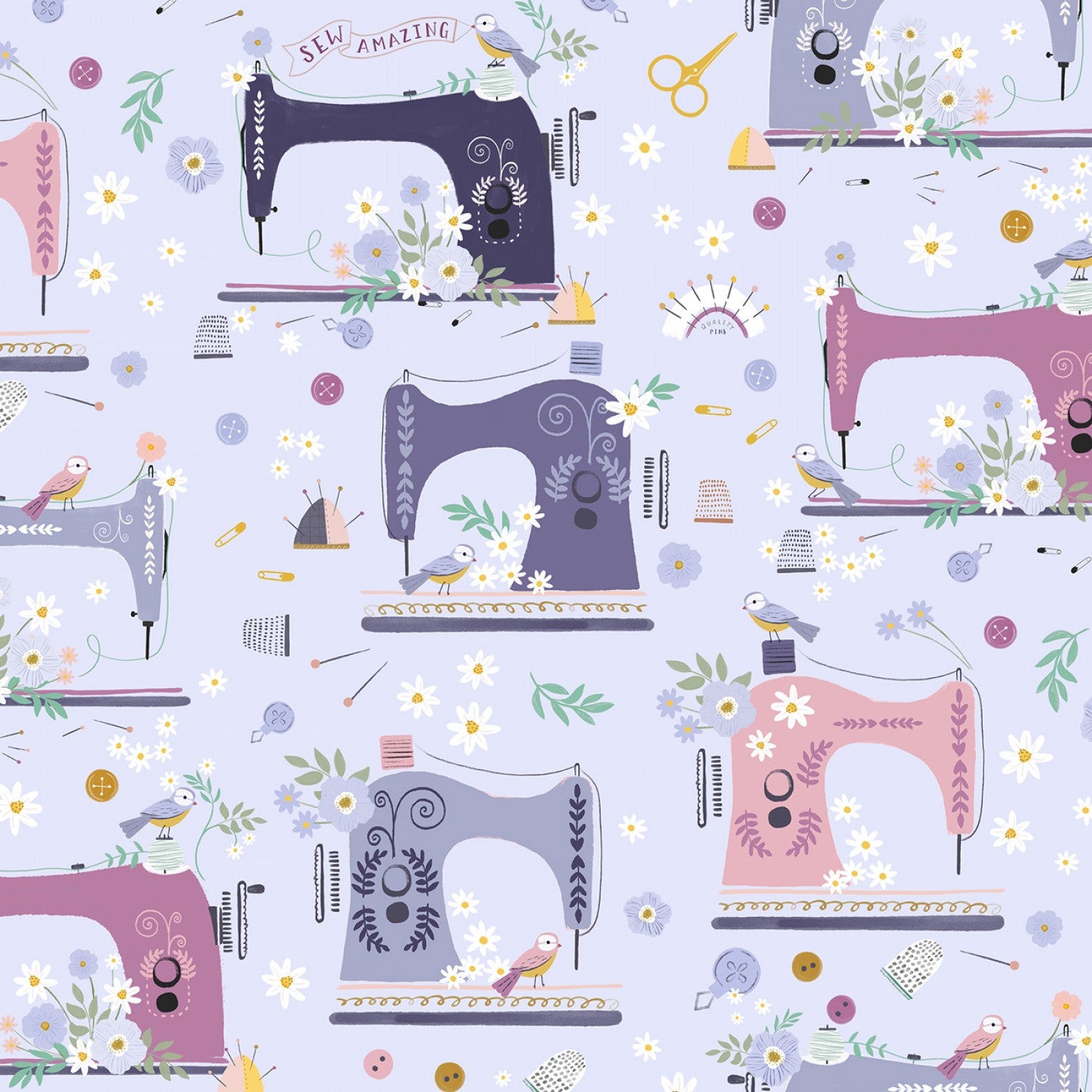The image is a repeat pattern wallpaper featuring whimsical illustrations of old-fashioned, hand-crank sewing machines in a cartoonish style. The sewing machines come in a variety of colors, including black, dark purple, gray, red, pink, and rose, and each is adorned with floral and leaf designs. Some of the machines also feature actual flowers as part of their motifs. Arranged against a lavender background, the sewing machines are interspersed with smaller symbols such as scissors, pins, pincushions, thimbles, thumbtacks, sewing needles, buttons, and leaves. Birds are also present; one bird is holding a banner with the words "Sew Amazing" at the top of the image. The overall aesthetic is reminiscent of festive wrapping paper or vintage-themed wallpaper, with a charming, nostalgic feel.